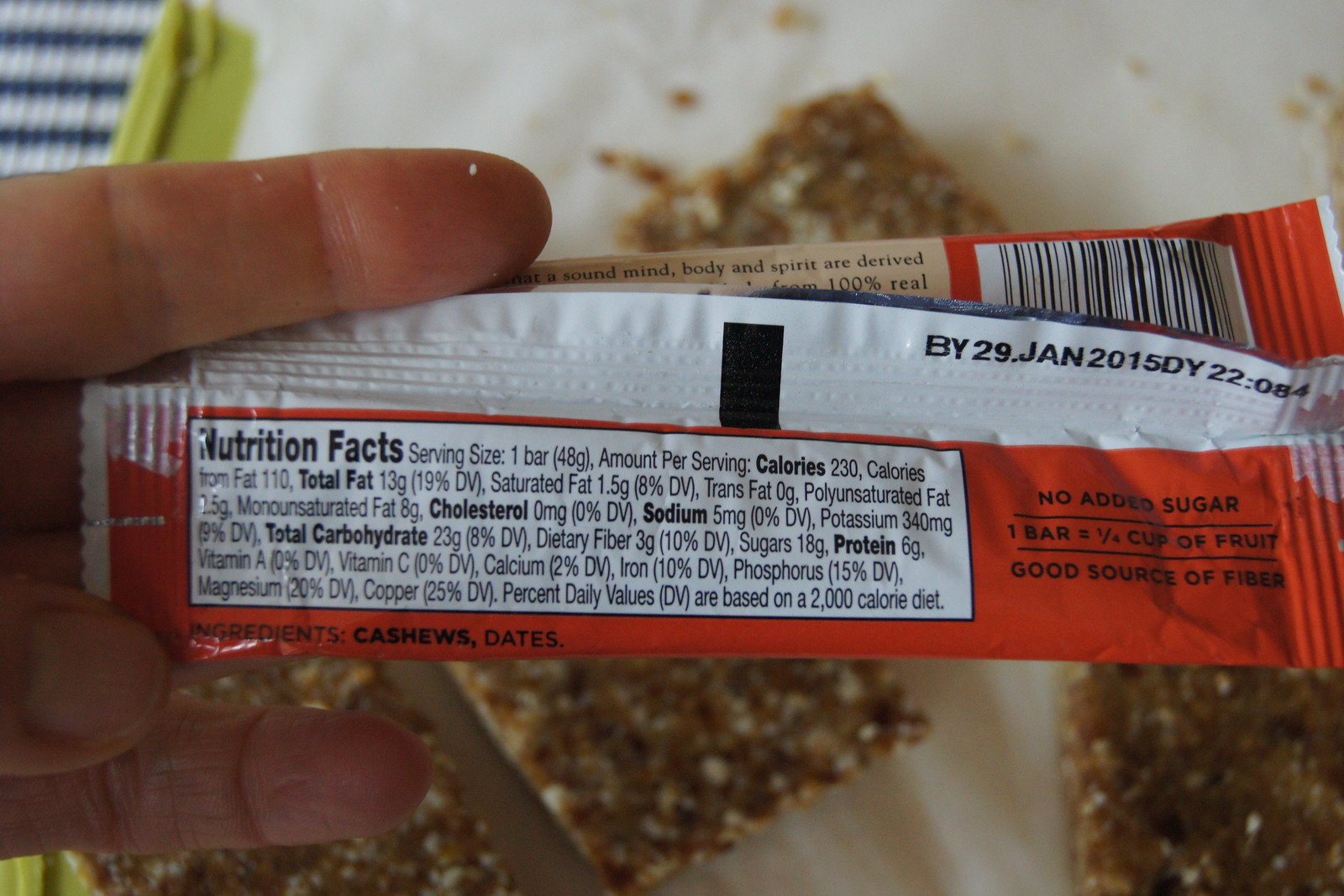In this image, a hand is prominently featured on the left side, with the fingers gripping a rectangular wrapper. The wrapper itself is predominantly red with a white back. Positioned at the top right of the wrapper, a black-and-white barcode is visible. Directly beneath the barcode, the text reads "buy 29.jan2015 dy22084." All the printed text on the wrapper is in black, including statements such as "No added sugar," "1 bar equals 1/4 cup of fruit," and "Good source of fiber."